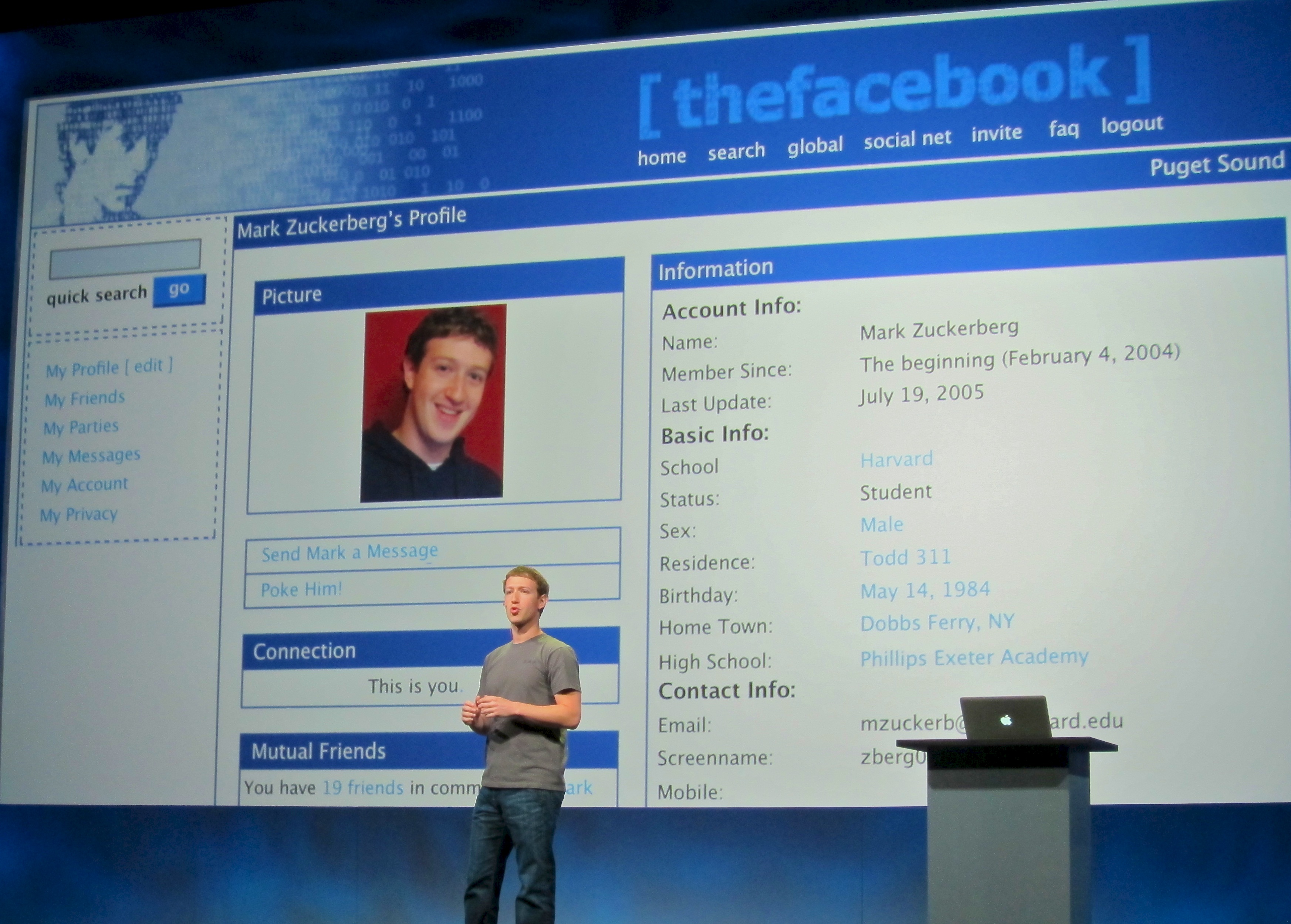This detailed photograph captures Mark Zuckerberg standing center stage, delivering a presentation about the early days of Facebook. He is dressed in his signature casual attire: a gray t-shirt and blue jeans. Positioned slightly left of center, he is actively engaging with his audience, gesturing with both hands as he speaks. To the right of the frame stands a gray podium with an open Apple laptop on top, although it appears that he is not using it directly during his talk.

The backdrop of his presentation is a prominent projection of an old-school Facebook profile page, distinctly labeled "thefacebook" in blue at the top. This early interface displays Mark Zuckerberg's own profile, replete with his photo and extensive personal information. The details include his name, account info showing he has been a member since February 4th, 2004, and his most recent update dated July 19th, 2005. Moreover, it lists his basic and contact information: Mark’s school (Harvard), student status, sex (male), residence (Todd 311), birthday (May 14th, 1984), hometown (Dobbs Ferry, New York), and high school (Phillips Exeter Academy). The profile also shows standard features of the early Facebook layout, including navigation options like home, search, global, social net, invite, FAQ, and log out.

In summary, this image encapsulates a moment from a pivotal presentation by Mark Zuckerberg, showcasing Facebook's initial user interface and emphasizing its college-oriented beginnings.